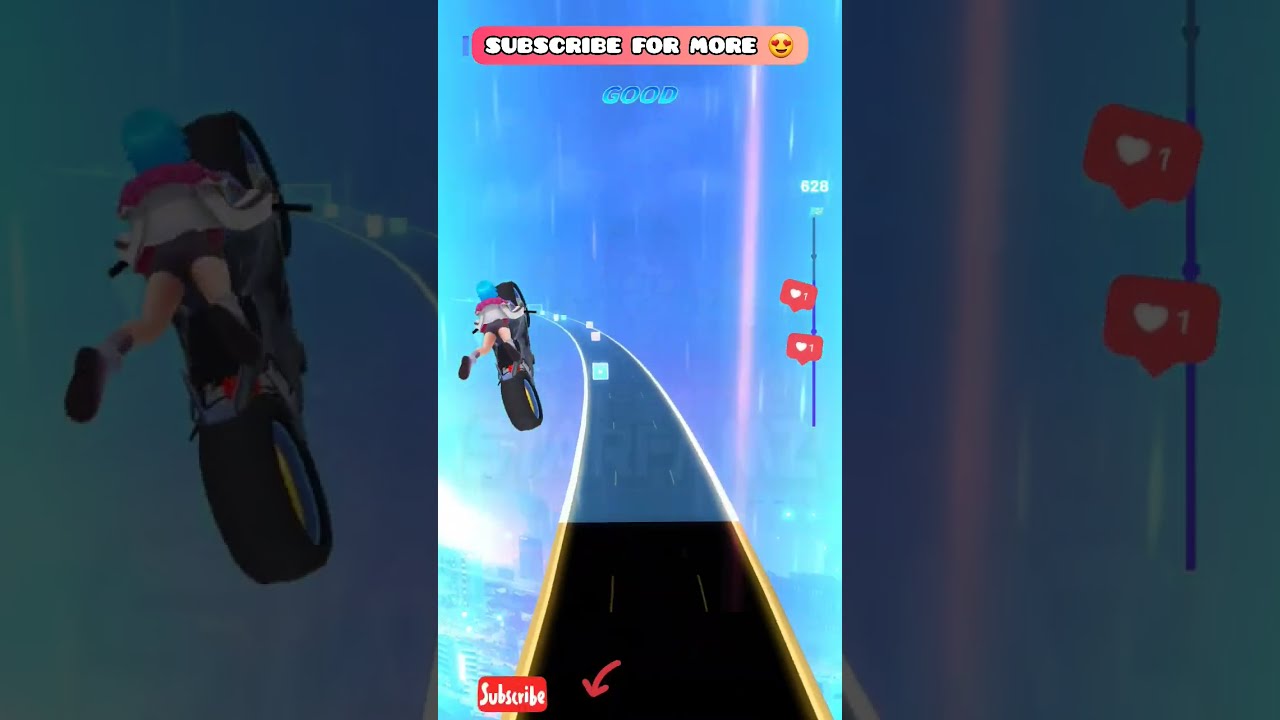In this vibrant screenshot from a video game, we see an animated, blue-haired character performing a daring motorcycle jump. The character, resembling a schoolgirl with a white top, pink cape, and dark shorts, is depicted mid-air with one leg off the bike, soaring above a black, three-lane road with yellow-highlighted edges. The background features a neon gradient of blues, purples, and pinks, adding to the dynamic nature of the scene. At the top of the screen, bold text reads "Subscribe for more" accompanied by a smiley emoji with heart-shaped eyes. There are also on-screen elements including a score of 628, the word "Good," and an icon indicating +1 likes. The bottom left corner features a red and white "Subscribe" button with an arrow, reinforcing the call-to-action for viewers.